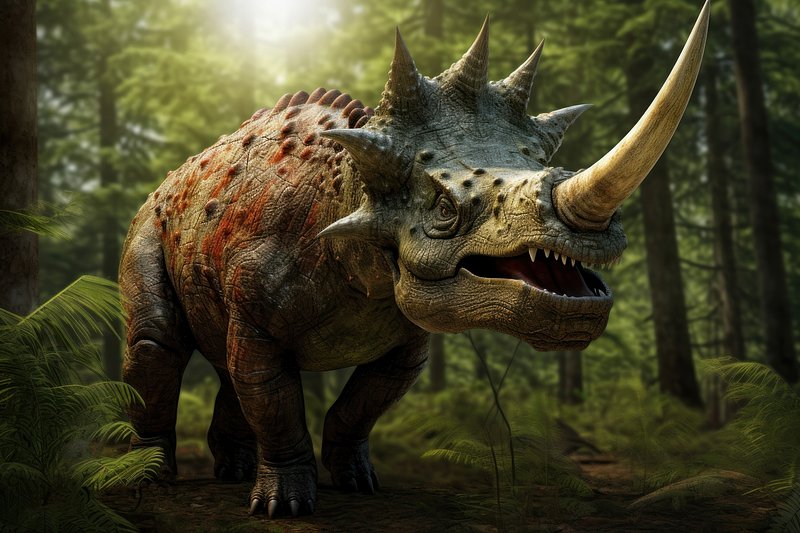This is a hyper-realistic, computer-generated image of a dinosaur standing in a lush, dense forest. The dinosaur, resembling a triceratops but with a single large, sharp white horn protruding from its nose, is vividly detailed with a blue-gray head and a tannish mouth and jaw. Its body features a striking blend of black with spots of orange and red, accompanied by raised bumps along its spine and face. The head is adorned with six spiky points in a circular arrangement. The dinosaur's mouth is slightly open, revealing sharp, spaced teeth. It stands on all fours on soil, surrounded by thin, tall trees and ferns. The image's high quality highlights the sunlight filtering from above, illuminating the scene and emphasizing the textures and colors of the dinosaur's skin. The creature appears to be front-facing but looking slightly to its left, with only one eye visible, creating a lifelike depiction of it in its natural environment.